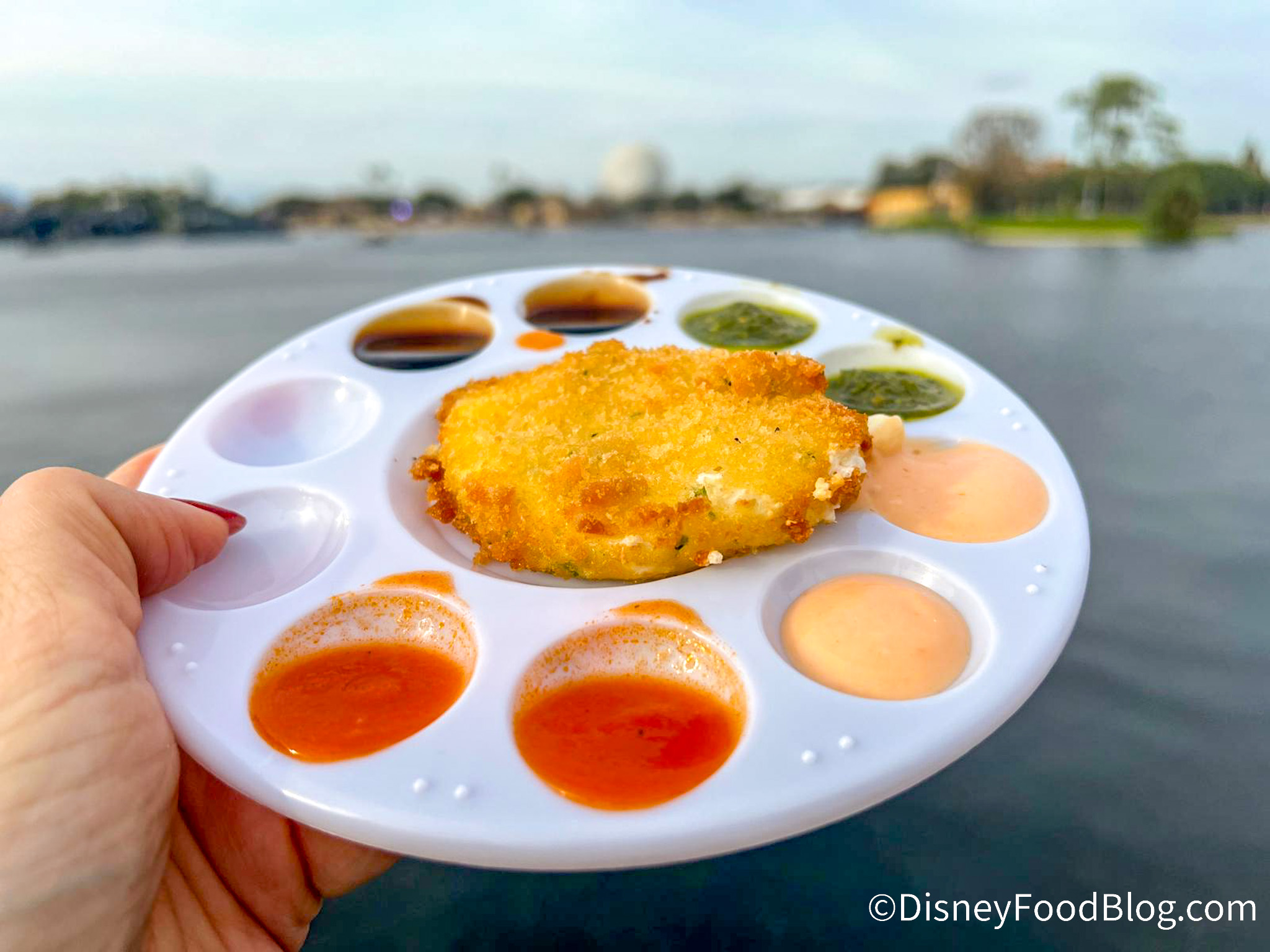In the foreground, a woman's hand with long artificial fingernails holds a uniquely designed plate resembling an artist's paint palette. The plate's central section contains a piece of breaded chicken, while around the edges of the palette there are ten small circular compartments, eight of which are filled with an array of dipping sauces. The sauces include honey mustard, barbecue, teriyaki, a see-through orange sauce akin to Buffalo or sweet and sour, a creamy orange sauce, and a green sauce, possibly avocado. The background is artistically blurred, revealing indistinct buildings, trees, and possibly a lake, suggesting an outdoor setting at Disney World, Florida. A watermark in the bottom right corner identifies the source as DisneyFoodBlog.com.